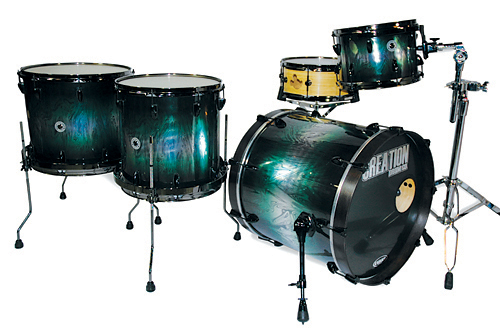This is an image of a five-piece drum set against a stark white background. The drum set has a shiny, gradient finish that transitions from a dark green at the ends to a lighter green and blue in the middle. The set consists of a bass drum positioned on its side, which features a mysterious white text that partially reads "REATON," with a yellow dot that might depict a sun or face. Two medium-sized toms and a snare drum share the same greenish-blue gradient color, and they are arranged closely together on the left. Additionally, there is one distinctly different drum with a yellow tint and black rim, mounted on its own stand to the side. The legs and attachments of the drum set are metallic and silver. The precise details of the text on the bass drum and the full nature of the design are difficult to discern.